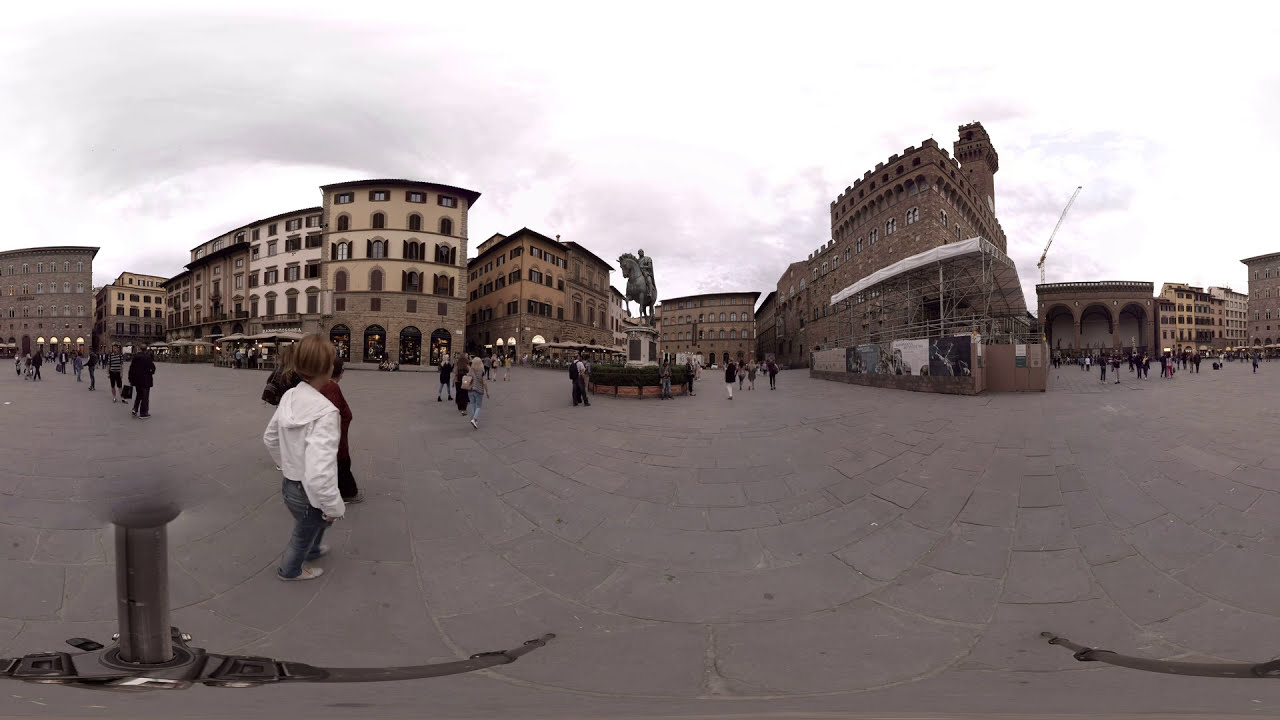This image captures a bustling, stone-paved plaza in a historic European city, taken during the daytime. The foreground displays dark gray stone blocks with scattered people dressed in casual clothing, including a woman in blue jeans and a white sweatshirt. Dominating the center of the plaza is a statue of a man riding a horse, set atop a tall, light-colored pedestal, possibly marble or granite. To the left, a row of multi-storied continental-style buildings features brick facades on the lower levels and yellowish plaster above, indicative of mid-century or older architecture. Some buildings show signs of renovation, with scaffolding and a crane actively at work. On the right side of the image stands a stone castle-like wall with large archways. The sky overhead is a grayish-white, dotted with clouds, adding to the charm and aged atmosphere of this European cityscape.